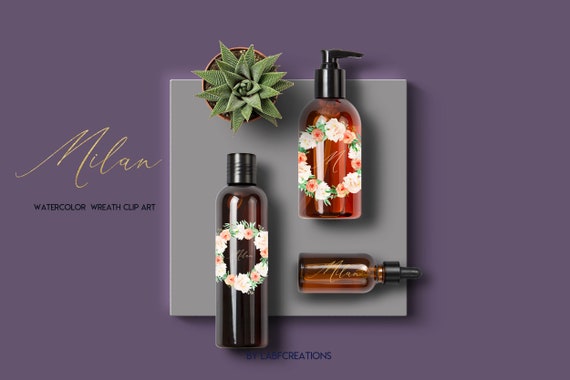This image is an advertisement featuring bath products on a purple background with gold and black text. The word "Milan" is written in cursive gold script, accompanied by the phrase "watercolor wreath clip art" in black print. The central focus is a light gray square with a drop shadow, showcasing an overhead perspective of four items. These include a succulent plant with radiating rosette-shaped leaves, a hand soap pump bottle adorned with a floral wreath of pink, white, and green flowers, a taller dark brown squeeze bottle featuring the same floral design, and a dropper bottle containing brown liquid, labeled "Milan" in matching script. Additional black text at the bottom also mentions "creations."